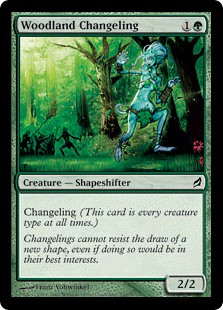This detailed Magic: The Gathering trading card is named "Woodland Changeling." It features a vibrant, graphic illustration of a blue-colored creature, described as a shapeshifter or changeling, running through a forest. The changeling is adorned with a fig leaf and has a distinctive tail. In the background, a group of three or four people, possibly wielding knives, can be seen in pursuit of the creature. The card's background also includes a prominent, large black tree at the center of the image, reinforcing the woodland setting.

The text on the card, in addition to its title, includes the description "Creature - Shapeshifter" and clarifies that the card has the Changeling ability, meaning it is "every creature type at all times." Further flavor text reads, "Changelings cannot resist the draw of a new shape, even if doing so would be in their best interest." The card's stats are shown as "2/2" in the bottom right-hand corner, and a tree logo is present in the top right-hand corner, signifying it as a green card.